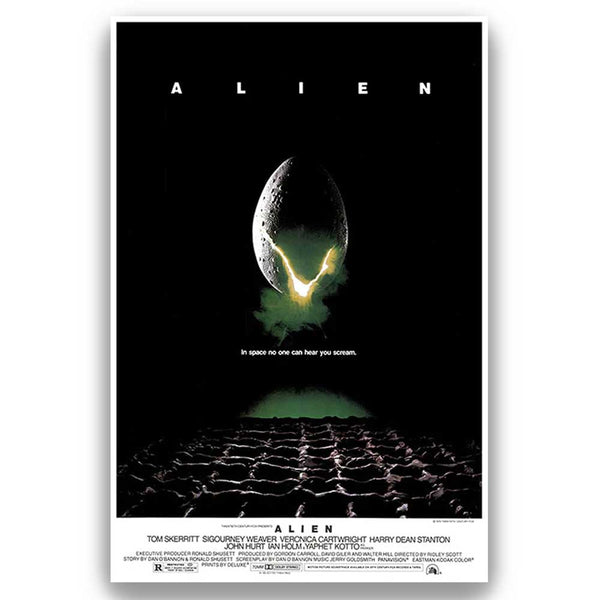The promotional poster for the original Alien movie features a stark black background framed by a slim white border. Dominating the top center is the title "Alien" rendered in pristine white text, capturing immediate attention. Prominently, in the middle of the poster, there is an iconic egg cloaked primarily in shadow, with a sliver illuminated from the left side, making the rest of the egg appear almost ominously dark. From the bottom of the egg, a V-shaped crack emits an eerie greenish-yellow light, adding to the sense of impending menace. Wisps of smoke or mist curl from underneath the egg, enhancing the ominous atmosphere. Below the egg, in small, almost indistinguishable font, the haunting tagline reads, "In space, no one can hear you scream." The poster subtly integrates names of the cast, such as Sigourney Weaver, Veronica Cartwright, and Harry Dean Stanton, along with production details, Dolby sound information, and the movie rating, all in a compact font at the bottom.